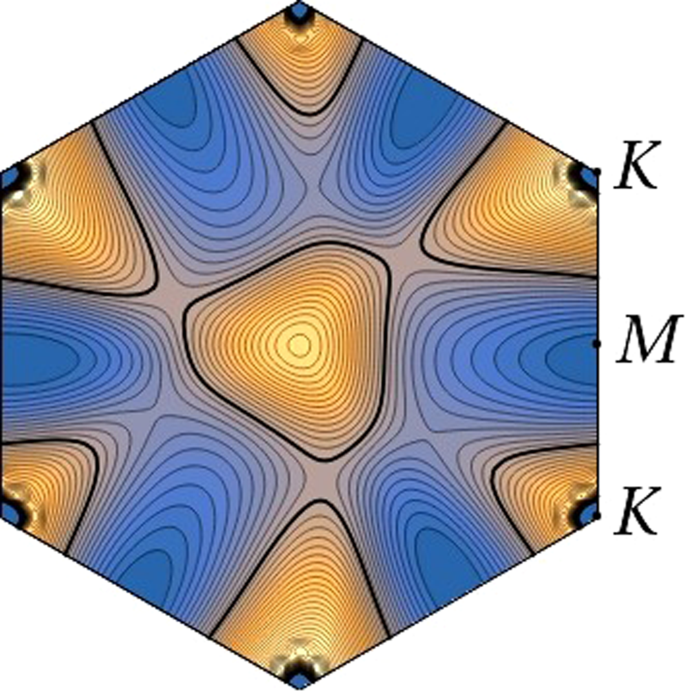The image depicts a hexagon with a trippy, psychedelic design characterized by intricate wave patterns and vivid colors. Each of the six edges of the hexagon is adorned with orange triangles, creating a striking outer border. Within the hexagon, the central section showcases a gold, wavy pattern resembling tree rings, bordered in black. Surrounding the center are alternating sections of blue and gold, giving it a kaleidoscope or flower-like appearance. The blue and gold areas are systematically outlined in black, enhancing their definition. On the right side of the hexagon, the bold black letters "KMK" are prominently featured, possibly indicating the creator of this mesmerizing artwork.